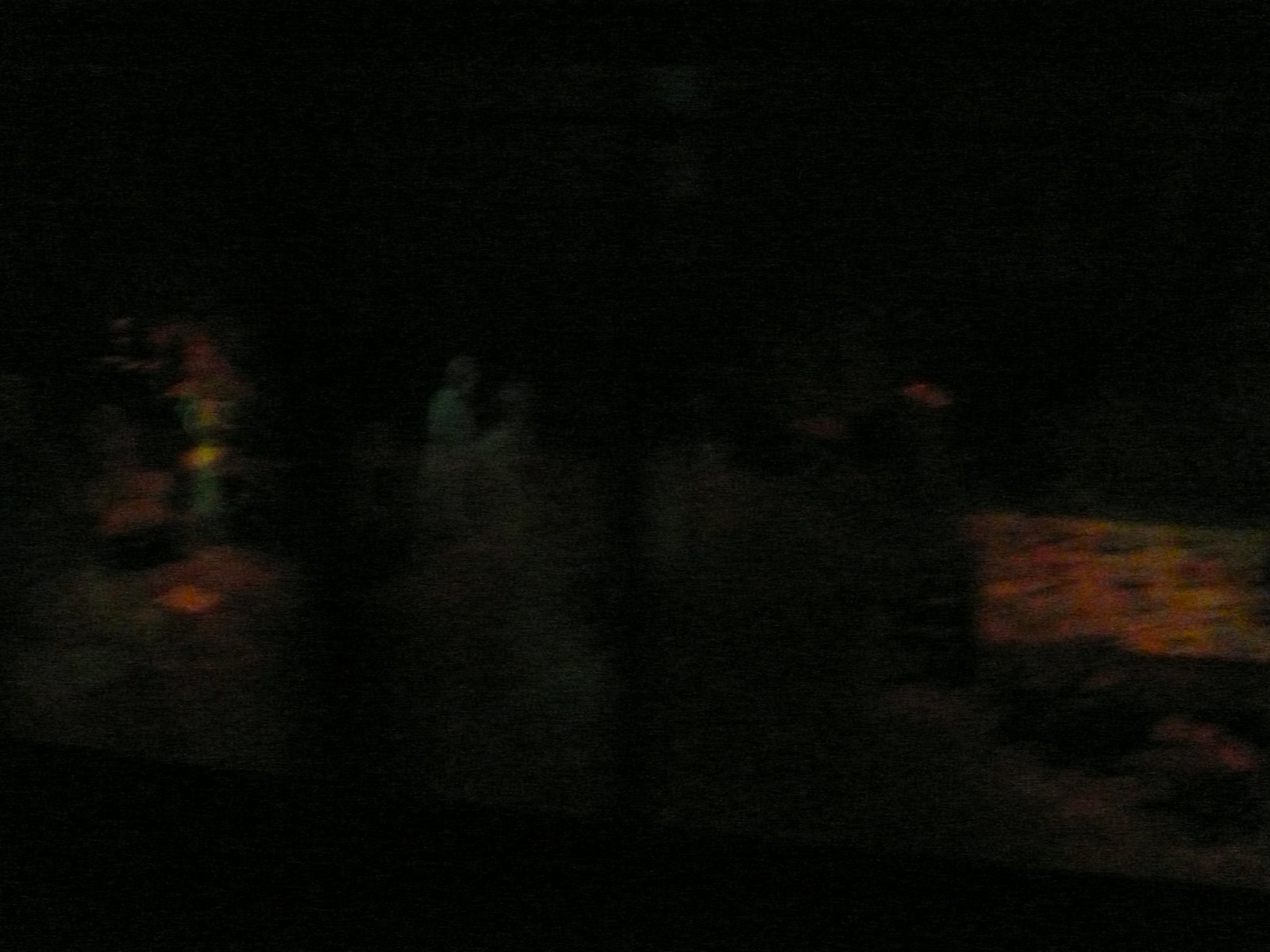In this image, the dark ambiance makes it challenging to distinguish objects clearly, though certain colors and shapes are discernible against the black background. On the left side, a muted and blurred scene appears to depict a room. Here, a red and black chair is noticeable, accompanied by a green cuckoo clock adjacent to its right. Near the bottom of this area, a small red square stands out. 

Moving towards the center, there seem to be two figures; their heads and bodies are vaguely visible, and they are enveloped in a white shading. Further to the right, there is some indistinct light gray shading. Near the center along the right edge of the image, a rectangle shaded in an interplay of green, black, yellow, and orange hues attracts attention.